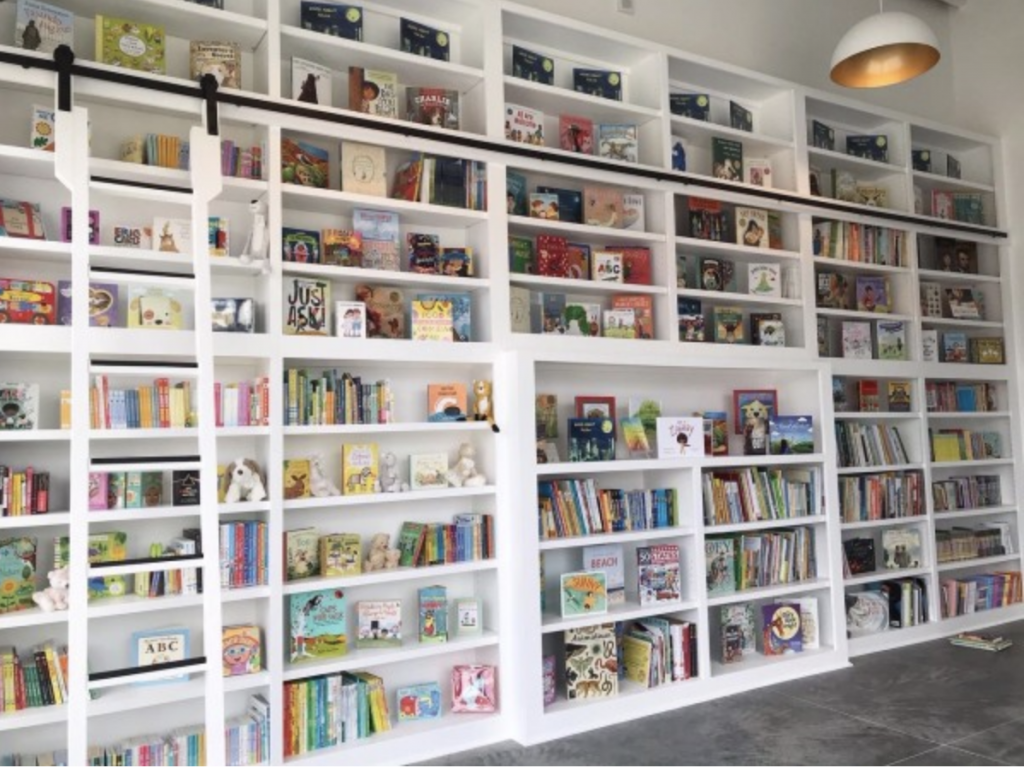The image captures a grand and meticulously organized children's library, featuring a colossal white bookshelf that spans the entire wall. The bookshelf, divided into multiple sections, contains six rows and six columns filled with a variety of colorful children's books and small stuffed animals, such as teddy bears. The top row of the bookshelf showcases 12 identical books neatly aligned, while other books are either displayed outward or positioned vertically with their spines visible. A white ladder with black steps and a sliding mechanism allows access to the upper shelves. The floor in front of the bookshelf is made of gray slate tiles, and a single book lies on the bottom right corner of the floor. Hanging from the ceiling is a white pendant light with a gold interior, casting a warm illumination over the well-organized and inviting space, perfect for young readers.